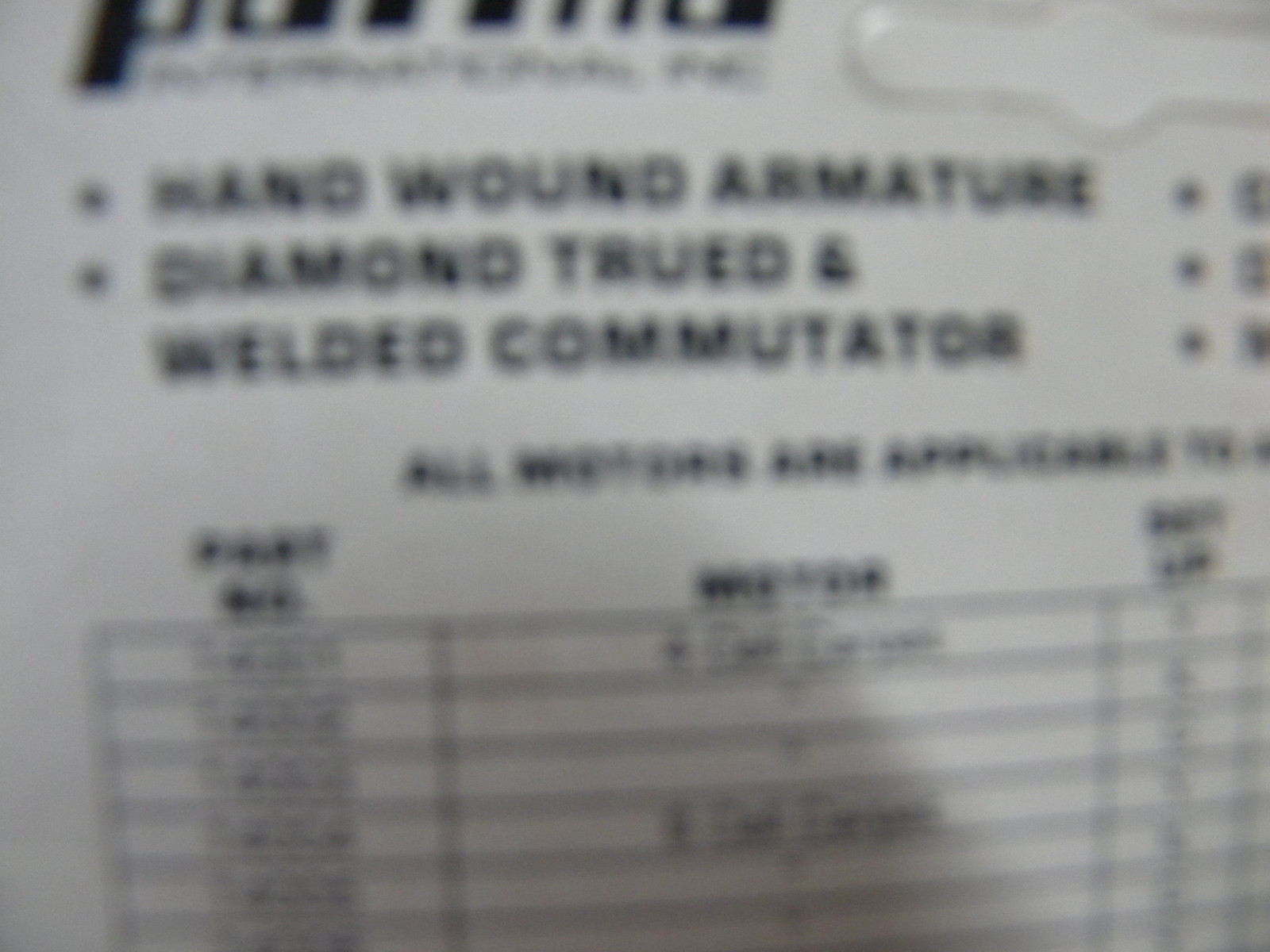The blurry image appears to be a label on some kind of packaging. Due to the distortion, it’s difficult to read the text with certainty. However, it seems to mention "wound armature" or "armatube" on the label. Towards the top, there is a partially visible logo beginning with the letter "P". Below the logo, there is a significant amount of writing. Near the bottom of the label, there's a box with lines, which might contain a list of ingredients or important information. Additionally, smaller print in columns suggests the inclusion of measurements or specifications.